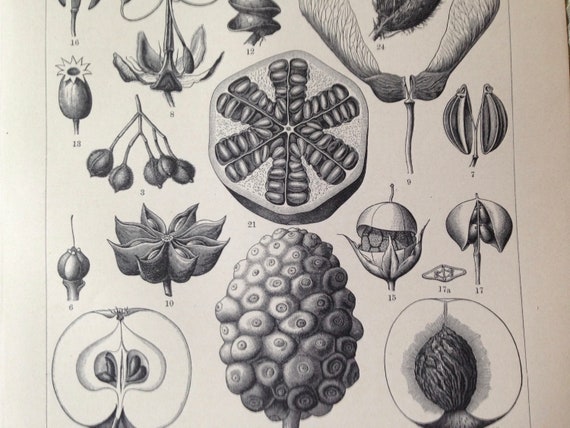The image depicts a vintage print of various fruit and vegetable seeds, illustrated in detailed black and white sketches on an old, yellowed paper. Central to the composition is a variety of cross-sections showcasing the seeds within their respective fruits. Notable examples include a halved apple and peach in the lower corners, both exposing their seeds and inner structures. Featured fruits range from familiar ones like apples, peaches, figs, and pomegranates to potential depictions of walnuts, pears, papayas, and star fruit. Some drawings also include the early blossom stages and unopened seeds, offering a comprehensive visual of the fruits' development stages. Each illustration is meticulously labeled with numbers, but no legend is available to further identify the items.